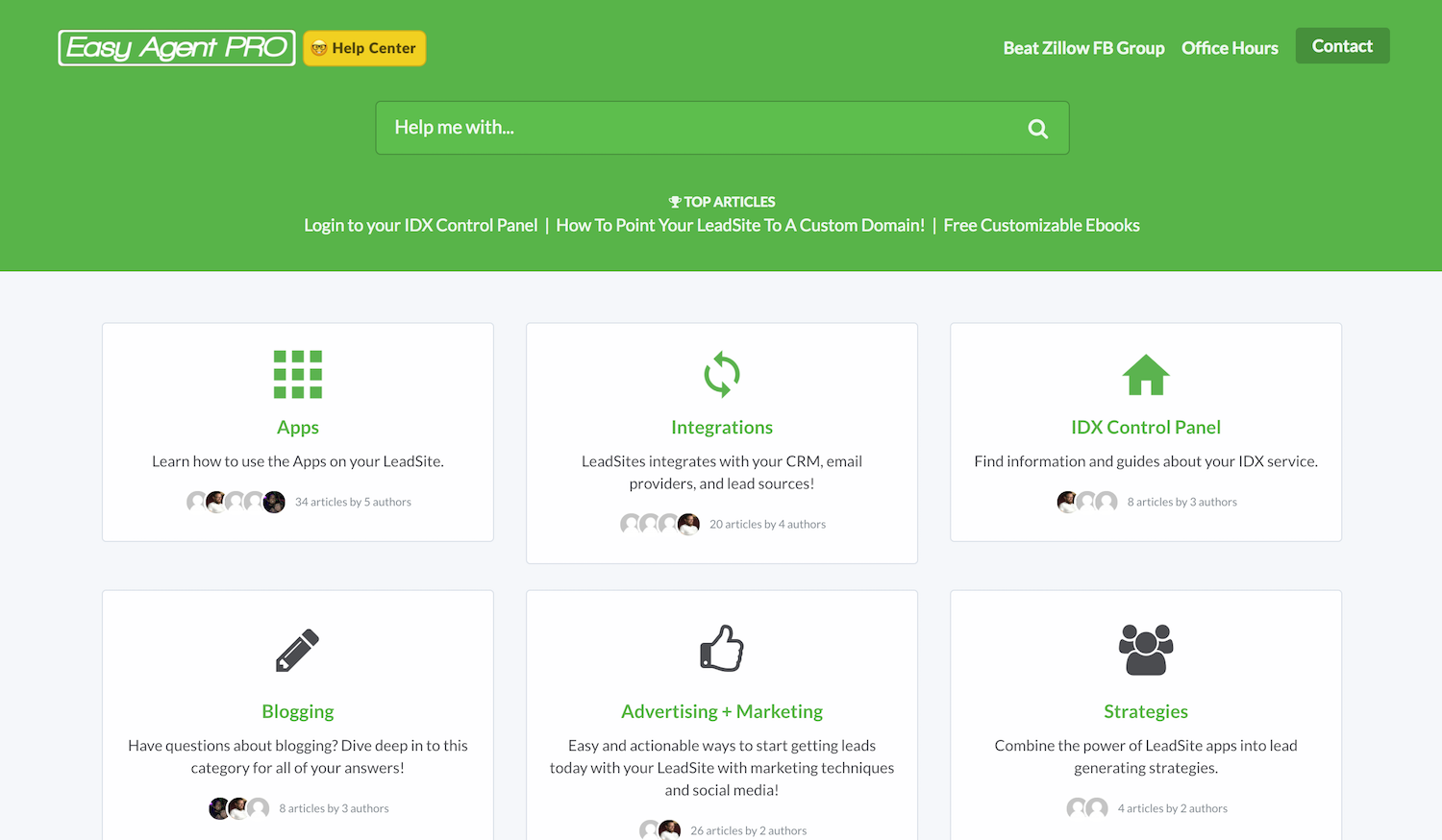This image appears to be a screenshot from the Easy Agent Pro website. At the top of the page, there's a prominent rectangular green banner. In the top left corner of this banner, the Easy Agent Pro logo is displayed. Adjacent to the logo is a distinct yellow button labeled "Help Center," featuring a smiley face adorned with sunglasses.

On the right side of the banner, there are links to "Best Zillow FB Group," "Office Hours," and "Contact," all of which are clickable for further navigation. Below the banner is a search bar with the placeholder text "Help Me With."

The page features several prominent sections. At the top, there are links to "Top Articles," including options for logging into your IDX control panel, instructions on pointing your lead site to a custom domain, and access to free customizable e-books. Each of these options is clickable.

Further down, the page is divided into six almost square but slightly rectangular areas. These sections include:

1. **Apps**: Information on how to utilize various apps on your lead site.
2. **Integrations**: Presumably details on integrating other services and tools with your lead site.
3. **IDX Control Panel**: Access to and instructions for using the IDX control panel.
4. **Blogging**: Resources and tools for blogging.
5. **Advertising & Marketing**: Guidance on advertising and marketing strategies.
6. **Strategies**: Various strategies to optimize the use of Easy Agent Pro services.

This organized layout ensures users can easily find and access the resources they need for effective real estate management and marketing.